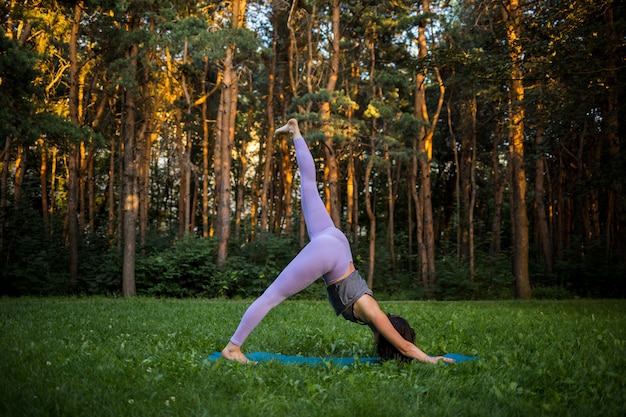A woman is captured practicing yoga outdoors on a turquoise yoga mat positioned in a grassy lawn within a wooded area. It's either early morning or late afternoon, as evidenced by the sharp angle of the sunlight creating dappled patterns through the trees. She is immersed in her routine, performing a challenging yoga pose with her head down, arms outstretched, and left leg elevated straight into the air while her right foot remains grounded. Her outfit includes purple yoga pants and a gray sleeveless athletic top, and her barefoot stance accentuates the natural setting. The background is filled with tree trunks and lush green leaves, with the lawn slightly elevating into a wooded area, infused with a mix of dark brown and green hues. The peaceful ambiance is set against a hint of blue sky, completing the serene outdoor scene.